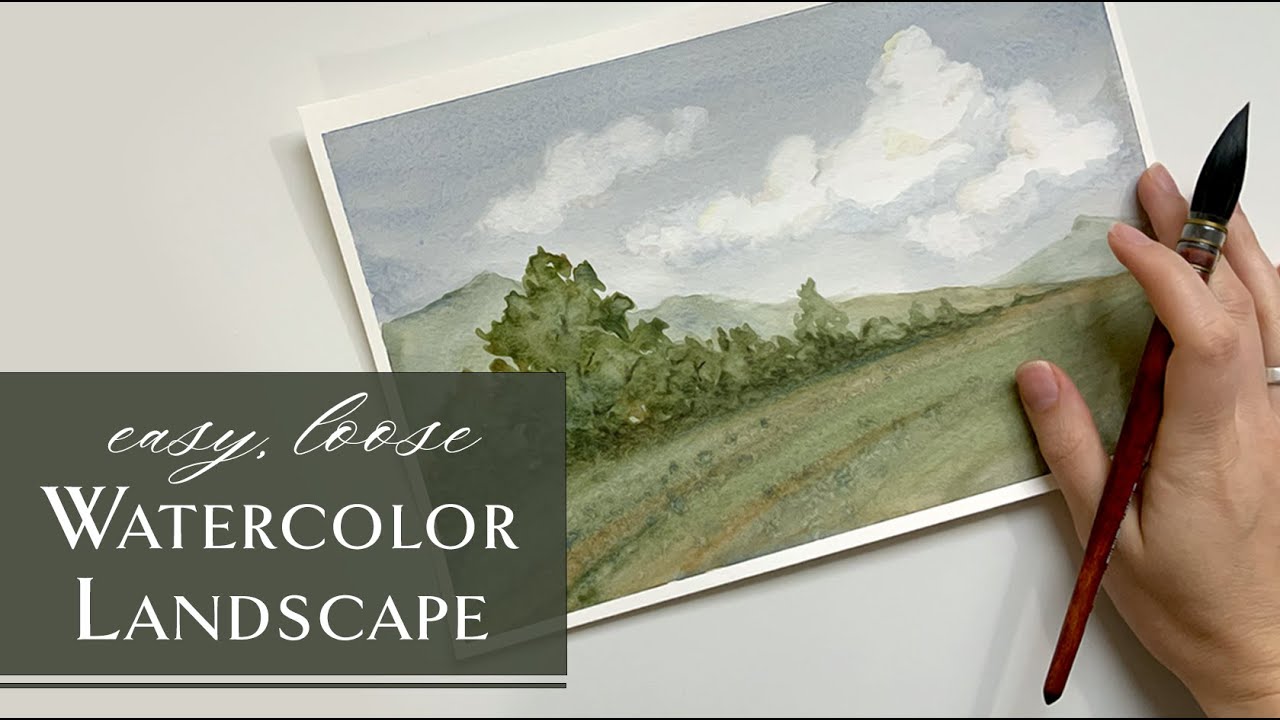The image appears to be an advertisement or a video thumbnail, featuring a detailed watercolor landscape painting on a rectangular white piece of paper with a subtle white border. The painting itself is a serene scene with a blue-gray sky filled with white clouds, sprawling greenery, and a field bordered by small trees, leading to distant, hazy light-green hills or mountains. To the right, a hand holds a thick wooden-handled paintbrush with black bristles, positioned delicately between the thumb, pointer finger, and middle finger. The background of the image is white, and a dark gray semi-transparent rectangle occupies the bottom left corner. Within this rectangle, the words "EASY, LOOSE" are written in white cursive at the top, and "WATERCOLOR LANDSCAPE" is displayed in larger white text below.